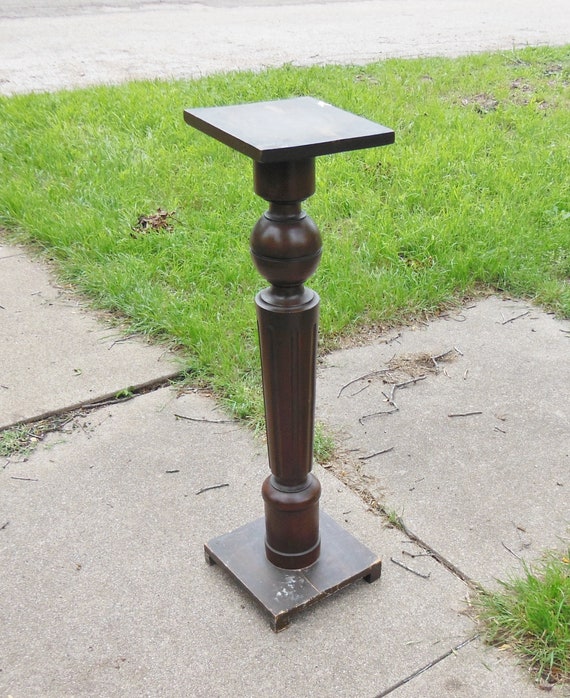The image captures an outdoor scene featuring a slightly worn, narrow pedestal made of very dark cherry wood, positioned on a cement sidewalk with visible concrete blocks and scattered twigs. The pedestal, potentially a tall wooden plant stand or a decorative column, has a square base and top, with intricate carvings in the middle section. Surrounding the pedestal is a slightly unkempt grassy area, and the background hints at a possible road. The scene might suggest a corner of a street due to the visible direction of the sidewalks. The pedestal appears to be the focal point of the image, standing prominently against the sidewalk squares.